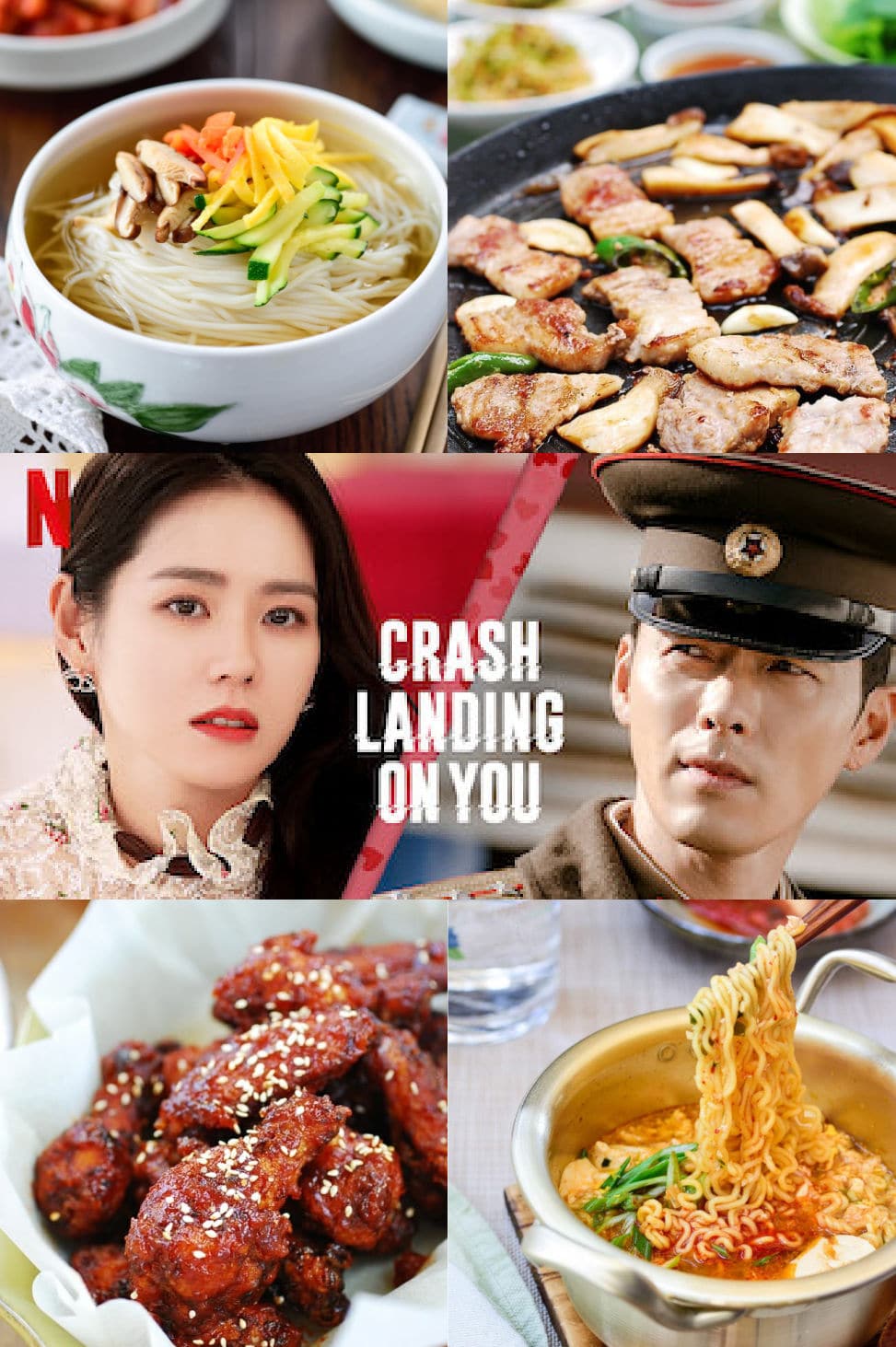This image is a promotional poster for the Netflix K-drama "Crash Landing on You." The main focus in the center is a picture of two characters from the show, indicating its connection to Netflix with an "N" logo. The characters, an Asian man in military attire and a woman, are prominently featured and occupy a space equivalent to two smaller images. Surrounding the central image are four different photographs showcasing a variety of Korean cuisine. 

At the top left, there is a bowl of noodles in a broth garnished with scallions or green onions and an egg. The top right features a dish of grilled meat sizzling in a skillet, accompanied by various vegetables including cucumbers. The bottom left image displays Korean fried chicken sprinkled with seeds, possibly sesame. To the bottom right, chopsticks are lifting noodles from a plate filled with broth and kimchi, creating a vibrant visual with colors like reds and yellows. Overall, the composition blends the allure of Korean food with the cultural appeal of a popular K-drama series, highlighting the rich colors and textures of both the cuisine and the show.